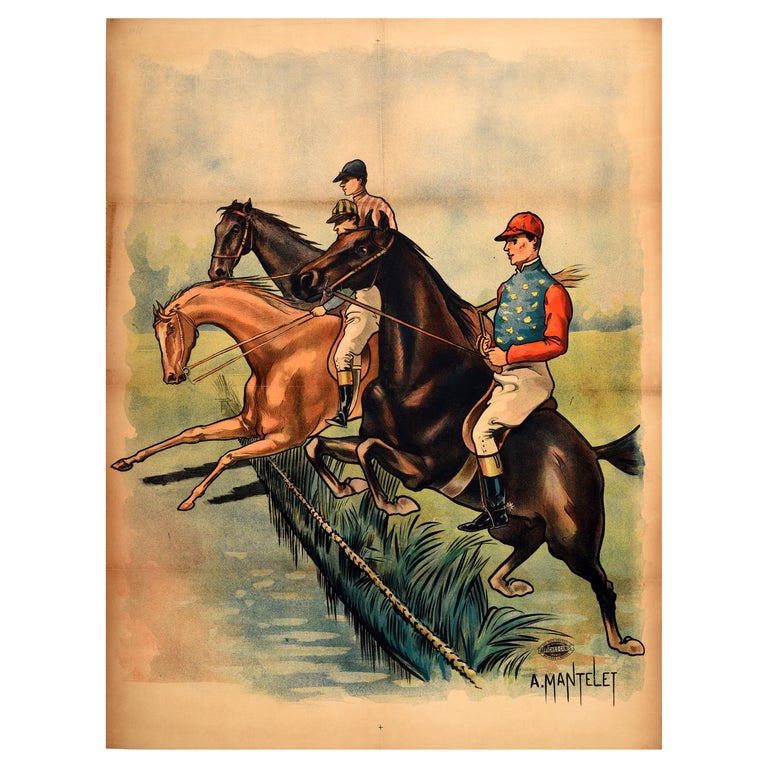The tall, rectangular painting by A. Mantelette, evident from the distinctive, overdrawn signature in the bottom right corner, depicts a dynamic scene of three equestrian riders mid-jump over a grassy barrier. The riders, each sporting distinct outfits, include the foremost jockey in a red cap, red long-sleeved shirt, a blue vest with yellow spots, beige-white pants, and black shoes with golden outlines, mounted on a dark brown horse. The central rider, obscured partially by the foremost horse, dons a blue shirt and sits atop a light brown horse that seems to lead the race. The rearmost jockey wears a blue cap and a vertically striped white and red shirt, riding a dark brown or nearly black horse. The backdrop features a watercolor blend of blues and greens, suggesting it's a daytime scene. The grassy field beneath the horses' hooves and the tall grass they are leaping over add to the vibrant, energetic atmosphere of the artwork.